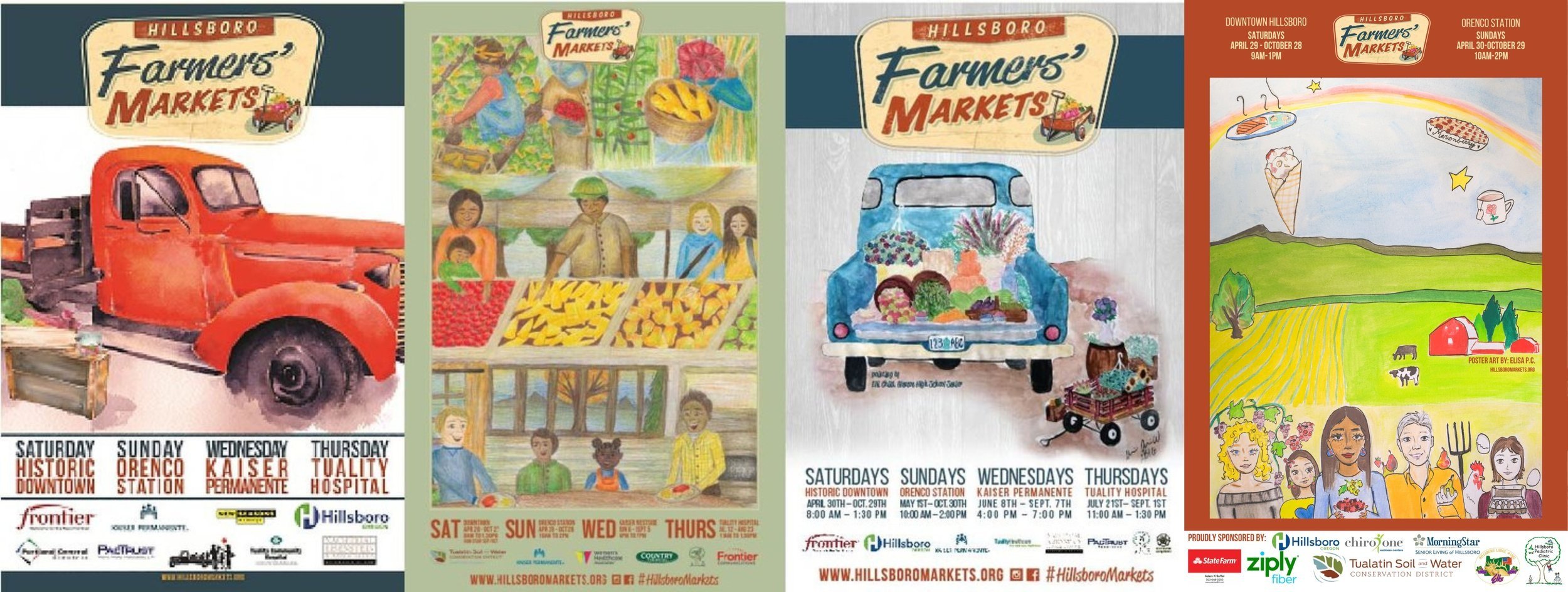The image features a series of four detailed advertisements for the Hillsboro Farmers Markets, each showcasing unique, hand-drawn artwork and specific event information. 

The first poster, predominantly blue and white, showcases a red pickup truck moving left to right across the top with the text "Hillsboro Farmers Markets" adjacent to a red wagon. Below, in blue and red lettering, it lists various market locations: "Saturday Historic Downtown, Sunday Dranco Station, Wednesday Kaiser Permanente, Thursday Tuality Hospital." Additionally, sponsor names in red, blue, yellow, and black are displayed at the bottom.

Adjacent to this is the second poster, highlighting "Hillsboro Farmers Markets" with a collage of four painted or penciled illustrations depicting produce and people of all ages. This poster also lists the market days and locations with similar sponsor acknowledgments.

The third advertisement features another pickup truck, this time blue and driving away from the viewer, filled with produce. Adjacent to the truck is a small wagon, with the market days and times noted below.

The final poster is a large, scenic farm drawing, featuring a red barn, green fern trees, a black and white cow, a brown cow, tilled farmland, and a tree at the edge. The sky is adorned with whimsical elements like an ice cream cone, a plate of food, a cup, and a star, all under a daytime setting. At the bottom, it depicts diverse individuals, including one with a pitchfork, alongside a chicken, reinforcing the community-centric vibe of the Hillsboro Farmers Markets.